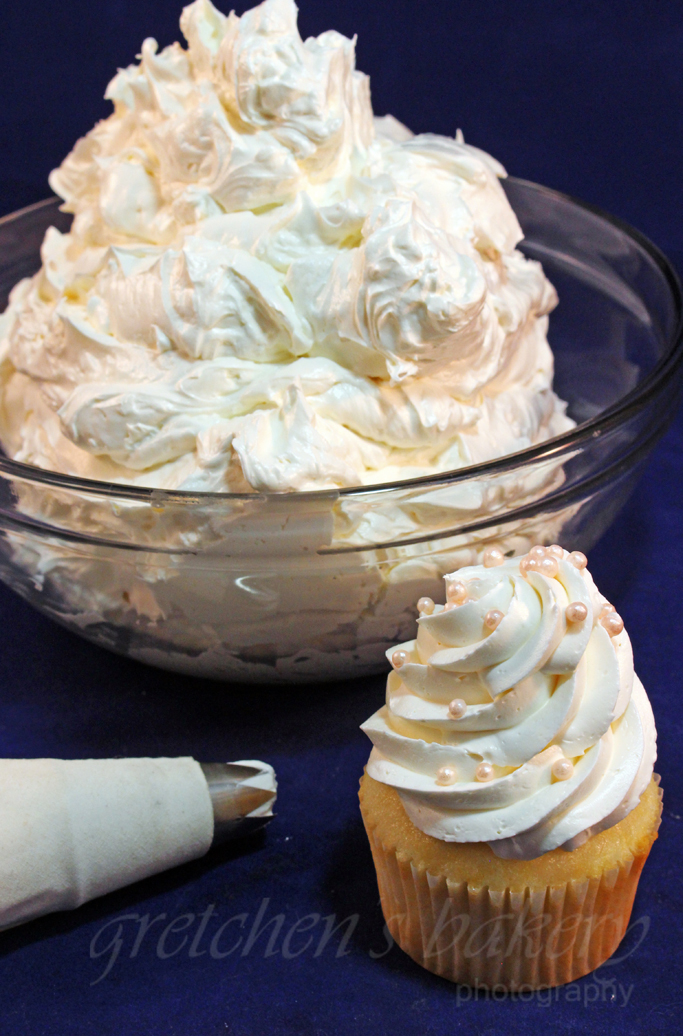This professional photograph features a close-up of a beautifully decorated cupcake and its accompanying tools, set against a striking blue background. Center stage is a clear glass bowl filled with an off-white icing that has a pinkish hue. Next to the bowl is a cupcake in a yellow wrapper, revealing the golden color of the cake beneath. The icing on the cupcake is artistically swirled and topped with delicate, edible pearls in a light orange, peach hue. To the left of the cupcake, a piping nozzle is visible, indicating the method used to apply the icing. The vibrant setup contrasts starkly with the background, enhancing the visual appeal. The image also bears a faint watermark at the bottom, reading "Gretchen's Bakery Photography," suggesting it may have been sourced from a professional website. The prominent colors in this composition are blue, yellow, white, pink, peach, and orange.